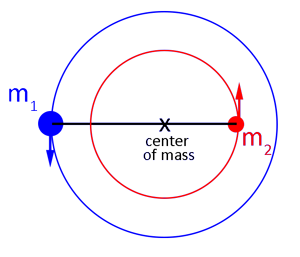The image is a detailed diagram featuring two concentric circles on a white background. The outer circle is blue and larger, while the inner circle is red and smaller. Both circles share the same center, labeled with an "X" that represents the center of mass. The blue circle has a large blue dot with a downward-pointing arrow at the nine o'clock position, labeled "M1." Similarly, the red circle has a slightly smaller red dot with an upward-pointing arrow, labeled "M2." A dark horizontal line connects the blue dot (M1) to the red dot (M2), indicating a possible relationship between these two points. This geometric drawing appears to illustrate a concept in mathematics or science, possibly related to mass distribution or equilibrium.